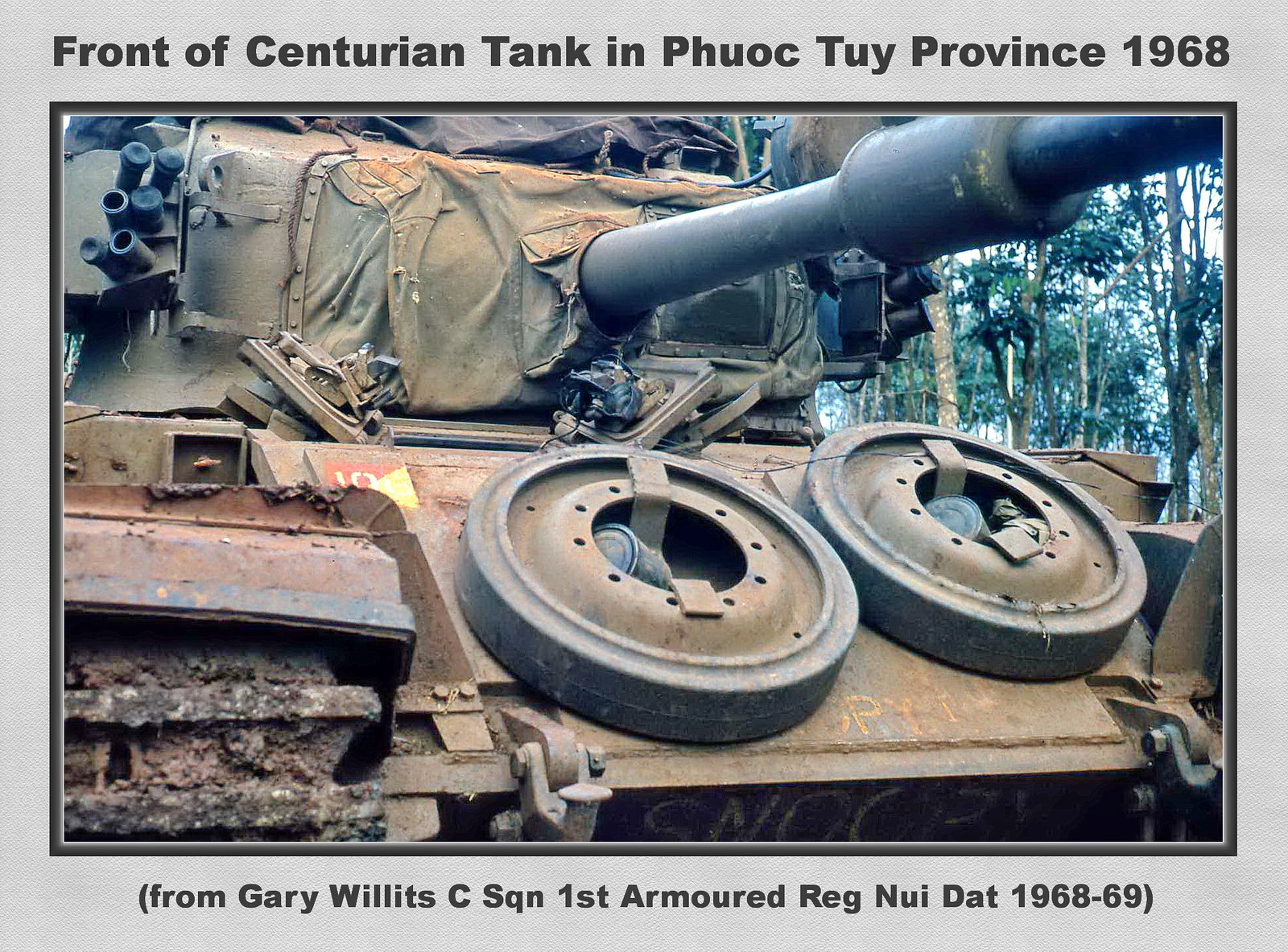This detailed landscape photograph captures a monumental Centurion tank situated in Phuoc Toi Province, Vietnam, during the Vietnam War in 1968. Dominating the foreground is the tank's main gun barrel, which extends prominently into the top right corner of the image. The tank itself is primarily a rusted brown, hinting at the wear and tear of active service, with patches of green paint still visible. A tarp encircles the base of the barrel, suggesting efforts to keep it dry.

In the left portion of the frame, one of the treads is visibly caked with mud, accentuating the rough terrain the tank has traversed. Two round objects, likely pulleys or wheels, are fixed to the vehicle, and several canisters are secured on the sides, possibly as spare parts. The tank's left side and top are draped in dark brown canvas materials, adding to its rugged appearance. On the top left, handwritten letters in yellow and white stand out amidst the worn metal, and a gray helmet rests just outside an open hatch, hinting at the human element of warfare.

The backdrop of the photo features numerous trees, providing a stark contrast to the mechanical behemoth in the foreground. The black label at the top of the image reads, "Front of Centurion Tank in Phuoc Toi Province, 1968," and the photo credit at the bottom attributes the image to Gary Willis from C Squadron, First Armored Regiment, 1968-1969. This caption provides a glimpse into the historical context and the imposing presence of the Centurion tank during the conflict.